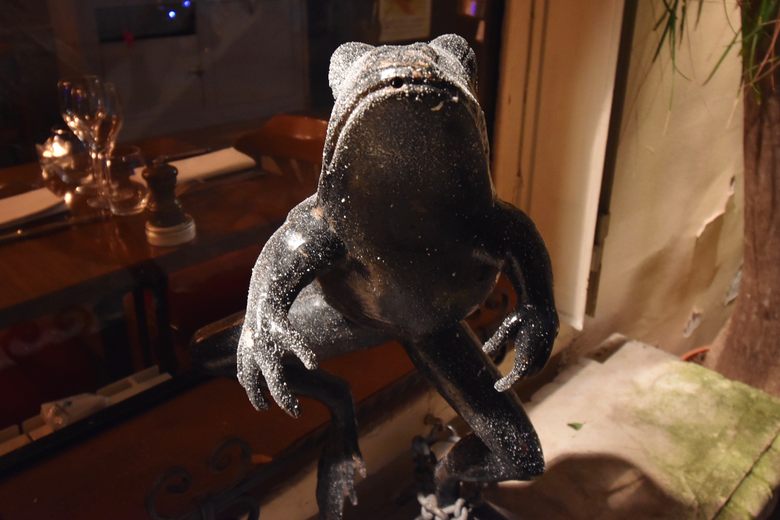This photograph, taken at night, depicts a weathered statue of a frog located in what appears to be someone's backyard. The frog, which could be made of metal or stone, features a rough, speckled texture and dark brown or black coloration, with white dust or powder scattered across its surface. The frog is captured in an unusual, almost anthropomorphic pose—standing on one leg as if mid-jump, with its front legs and long feet positioned as if preparing to grab something. Its large, bulbous eyes, which pop out from the top of its head, are notable, though partially obscured in the dim lighting. A chain is wrapped around the statue, possibly as a security measure to prevent theft.

In the background, you can see glimpses of a wooden table piled with miscellaneous items and a partly visible chair. To the right of the statue, there is some moss and a plant hanging from the ceiling. Peeling white wallpaper and a tree trunk with some green foliage further indicate that this scene is set outdoors, possibly on someone's property where visitors can easily access the area. The entire scene is dimly lit by an overhead light source, casting soft shadows and highlighting the frog statue as the focal point of the image.